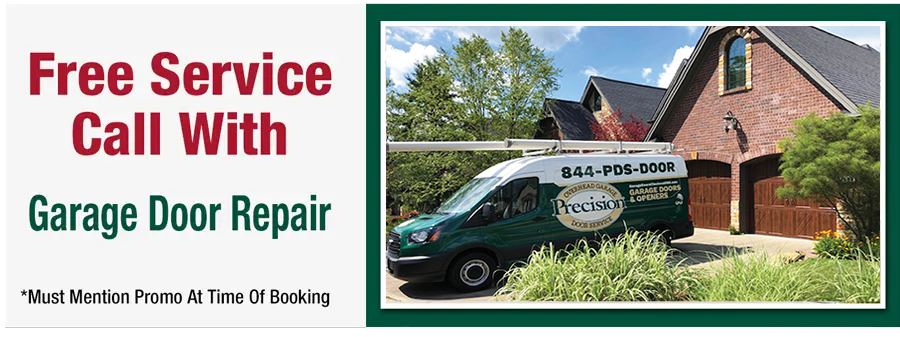**Caption:**

This advertisement features a horizontally-oriented layout. On the left side, set against a gray background, is bold red text stating, "Free Service Call With," followed by green text reading, "Garage Door Repair." Beneath this, it specifies, "Must mention promo at time of booking," with an asterisk indicating that this must be mentioned to avail the free service call.

The right-hand side of the advertisement displays an image bordered in green, with a white border inside the green frame. The image captures a service vehicle—a white van with a dark green lower half and emblazoned with the phone number 844-PDS-DOOR. The van, parked in a driveway surrounded by green bushes, is branded with "Garage Doors and Openers," "Precision Door Service," and "Overhead Garage." The backdrop includes a red brick building with two wooden garage doors, adding context to the garage door repair service being advertised.